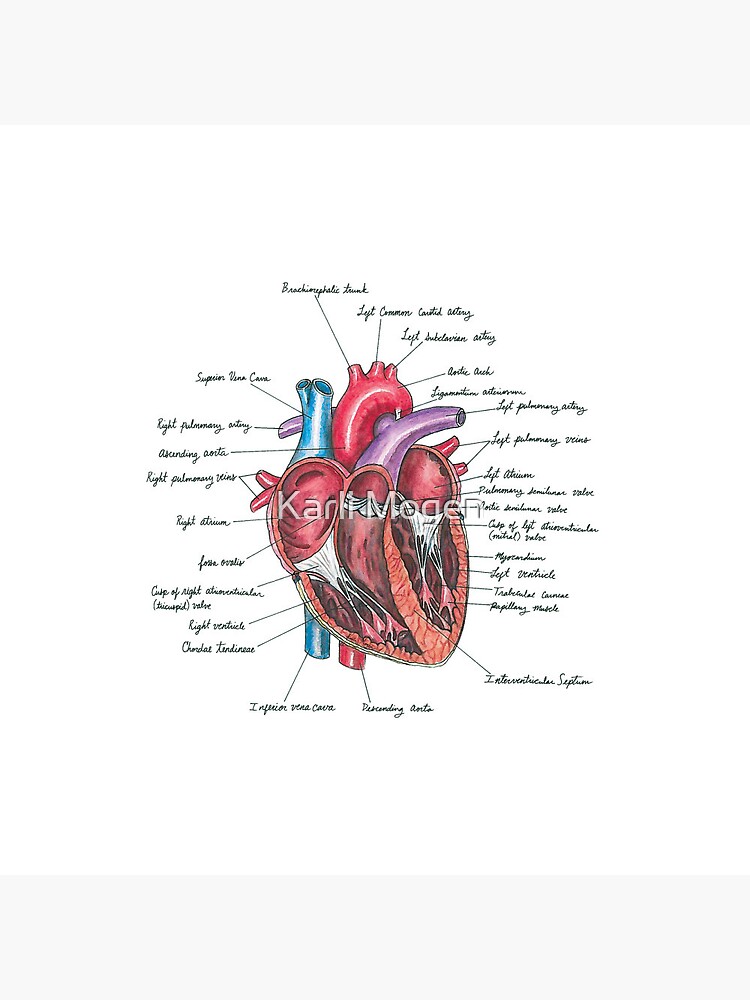This is a highly detailed anatomical drawing of a human heart in cross-section, created with colored pencils. The heart is rendered in vivid shades of red, blue, purple, and gray, with accents of white and light pink to highlight different anatomical features. Each part of the heart is meticulously labeled in black cursive script, with lines connecting the labels to their corresponding regions. Notable parts such as the left atrium, left ventricle, interventricular septum, right atrium, right ventricle, and a variety of arteries and veins are clearly marked. In the middle of the heart, the name "Carl Mogen" is inscribed in white, prominently across the illustration. The blend of colors and precision in labeling makes this anatomical drawing both educational and visually engaging.